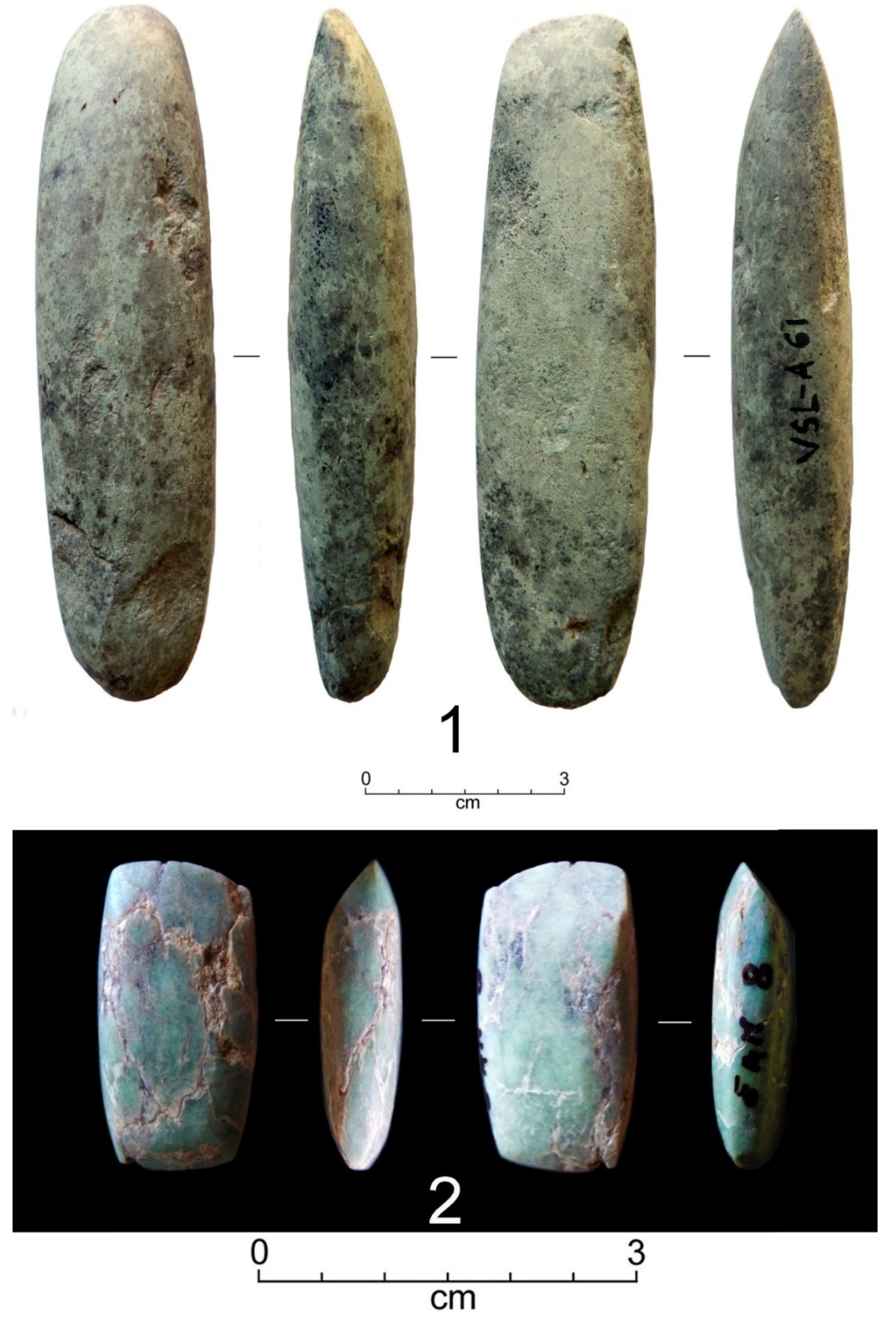This image showcases two sets of ancient stone tools, likely axe heads, arranged vertically in a portrait orientation. The top part, occupying approximately 75% of the image, features four elongated, oval-shaped stones, mostly gray with some shades of black, purple, and white. These stones are sequentially rotated to display different angles and have "VSL-A67" inscribed on them in permanent marker. Below these stones is the label "1" accompanied by a centimeter scale measuring their length from 0 to 3 cm.

In the bottom quarter of the image, against a black background, are four stones with different shapes: the first and third are rectangular, while the second and fourth are more oval with pointed ends. These stones are primarily light brown and turquoise, interspersed with purple and off-white cracks. Similarly, the stones are labeled "2" with a centimeter scale from 0 to 3 cm. An inscription "F AM 8" is visible on the last stone of the second set, though it is somewhat obscured.